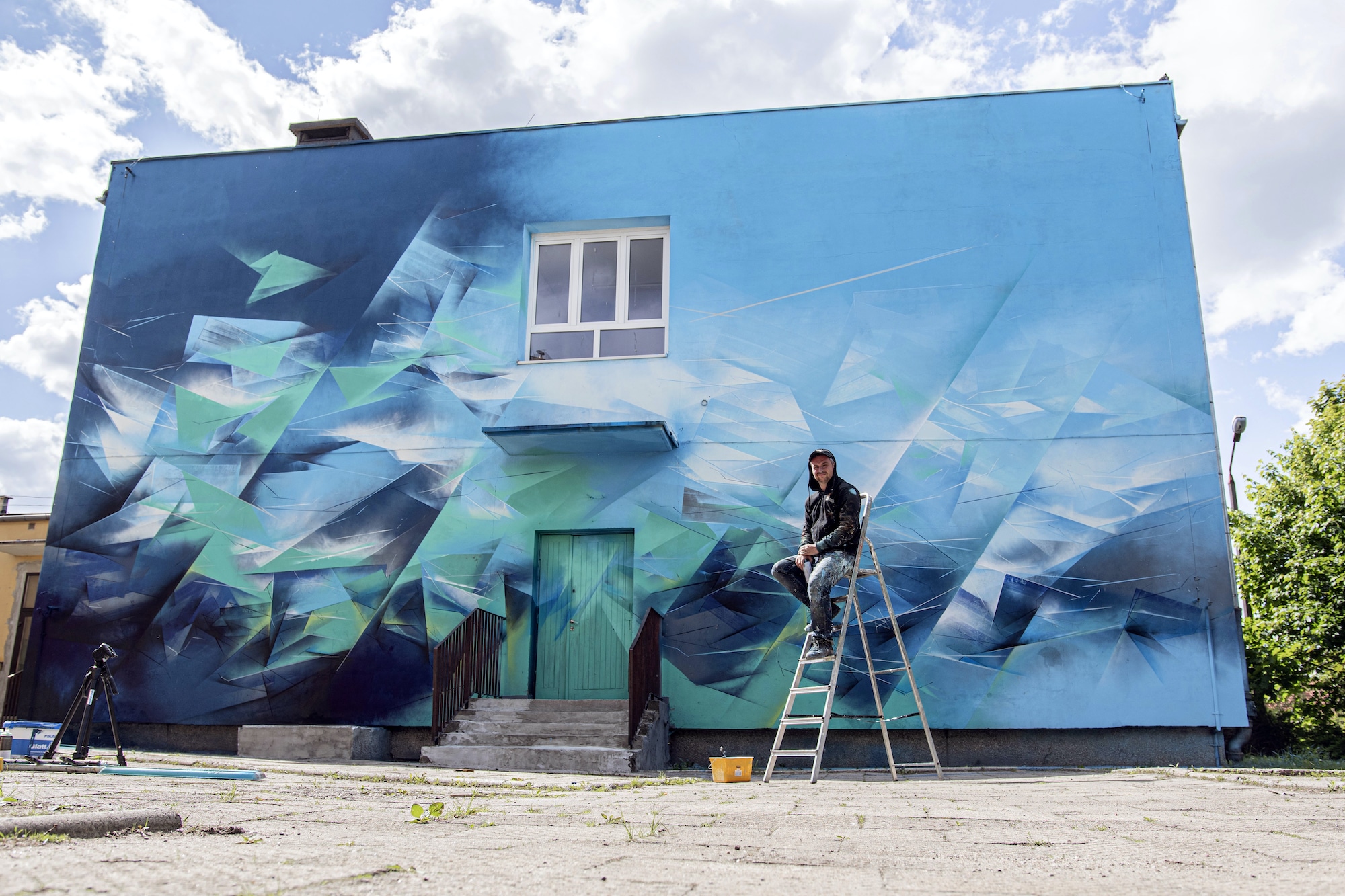This rectangular photograph, taken outdoors on a sunny day, captures a vibrant scene dominated by a uniquely painted boxy building. The bottom of the image shows a cement paver ground leading to the central building. The structure features five cement steps with metal guardrails on either side, leading up to a green door. A man with light skin, wearing a black jacket with a hood or hat and blue jeans, is perched on a silver ladder to the right of the guardrail, smiling at the camera.

The building behind him is strikingly painted with a fractal-like, geometric design. The color scheme transitions from light blue on the upper right to a mix of white, green, and dark blue towards the bottom and left, culminating in dark navy blue at the corners. Above the door, there is a small overhang providing shade, and a single window with five panes of glass and a white grid is situated above it.

To the right of the building is a green bush, while another building is visible in the background to the left. The foreground contains various items, including a camera on a tripod, some boxes, and a yellow basket, suggesting a scene of active work. The backdrop reveals a vibrant blue sky filled with thick white clouds, with additional trees and buildings visible, enhancing the dynamic outdoor setting.